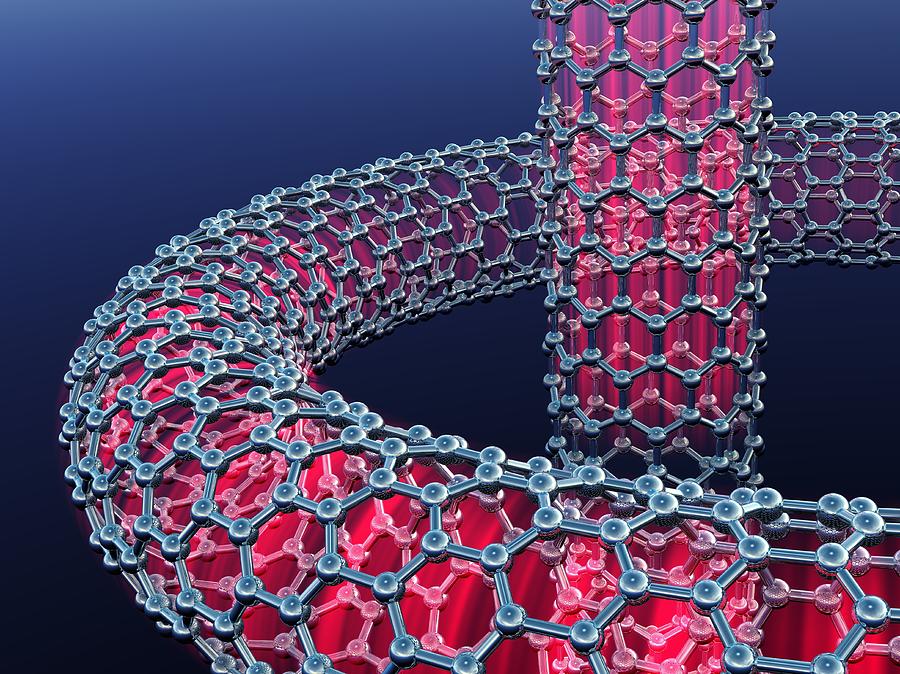The image resembles a detailed illustration reminiscent of diagrams commonly seen in a chemistry class, specifically resembling a DNA structure. It portrays two spiral strands akin to ropes, curving from right to left and suggesting the form of a DNA helix. Although the complete helix isn't visible, it appears as if part of it extends into a circular shape, of which only a semicircle is shown.

In the foreground is a prominent, snake-like strand meandering vertically between the semicircular helix. The image features numerous blue octagonal shapes, which appear to be wrapping around an internal fuchsia-colored structure. These blue octagons are interconnected by small circular elements, creating a complex and intertwined pattern atop the fuchsia material. The overall aesthetic gives an impression of intricately linked components, reminiscent of molecular structures.